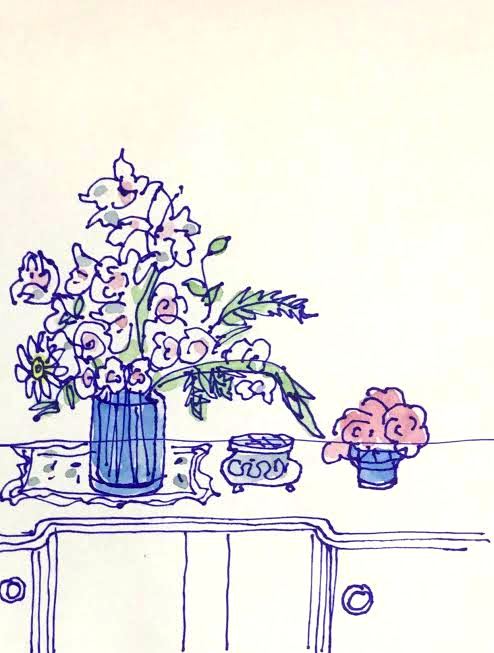The image is a detailed drawing on ivory-colored, off-white paper that transitions from yellow to white at the top. The scene depicts a still life arrangement on a rectangular vanity or counter surface, which features two front-facing cabinet doors with round knobs. On the left side of the surface, there is an ornate tray with scalloped edges, holding a blue vase filled with an elaborate bouquet. The bouquet features light watercolor shades of pink and blue, with green foliage, including roses, daisies, and lilies. To the right of the vase is a small blue teacup with a white pattern and next to it, a diminutive pot with three visible pink roses. The drawing employs an ink line technique accentuated by watercolor highlights, lending a delicate and vibrant touch to the floral elements and surface objects.